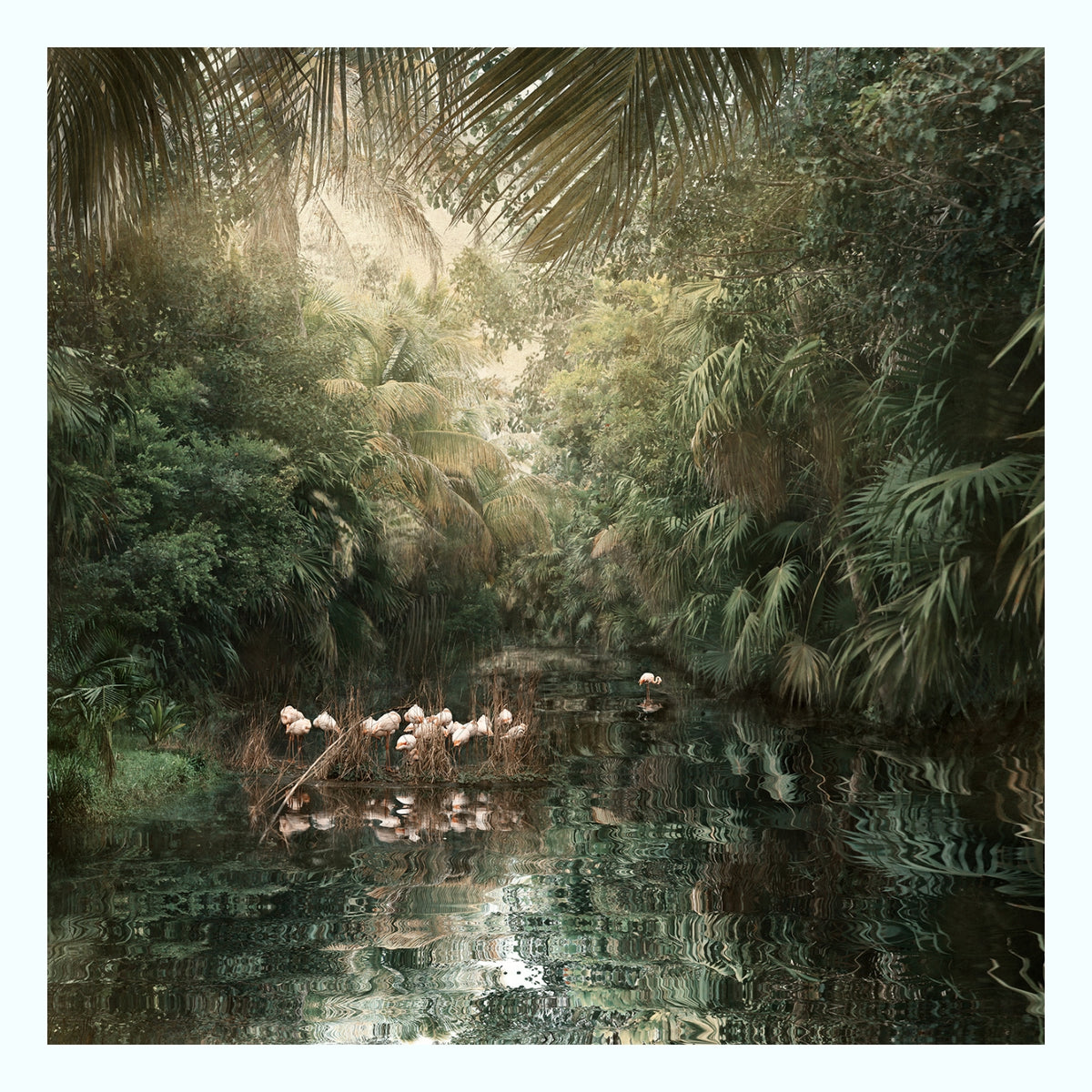This is a highly detailed and vibrant photograph capturing the serene beauty of a dense jungle setting during mid-afternoon. The image features a rippling river or pond flowing through the center, with numerous overgrown trees and ferns lining its banks. The waterway, which appears bluish-green and reflective, mirrors the thick green canopy above. The sun penetrates through the treetops, casting a mixture of green, brown, yellow, and white hues throughout the scene.

Amidst this lush landscape, approximately a dozen flamingos stand in the middle ground, some of them with their heads dipped into the water, presumably searching for food among the dry reeds and small aquatic plants. A single flamingo is isolated in the background, adding depth to the scene. The presence of numerous reeds, various other plants growing out of the river, and patches of orange where some leaves have dried, further enhance the natural richness of the environment. The overall impression is that of a tranquil, overgrown rainforest, teeming with life and vibrancy.